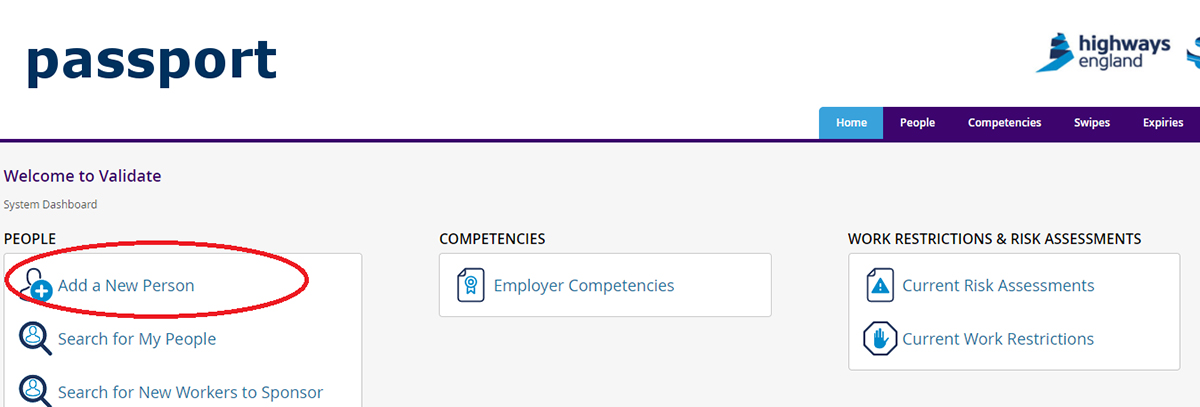The image shows a webpage from the Highways England website. In the upper right-hand corner, the Highways England logo is displayed in shades of blue. On the far left, the word "Passport" is prominently written in large blue font. Just below "Passport," in purple text, it reads "Welcome to Validate." 

In the central section of the page, a red circle highlights the "People" category. Within this category, three options are presented, and "Add a New Person" is emphasized with a red circle around it. To the right, the next column is labeled "Competencies," which contains a clickable header titled "Employer Competencies." The third column is "Work Restrictions and Risk Assessments," which lists two clickable options: "Current Risk Assessments" and "Current Work Restrictions."

Near the top of the webpage, there are four purple navigation bars, with the "Home" bar distinguished in light blue. The overall background of the webpage is a clean, solid white, with the aforementioned blue, purple, red, and black elements providing contrast and highlighting key sections. The design is straightforward, with no additional landscaping or background imagery.